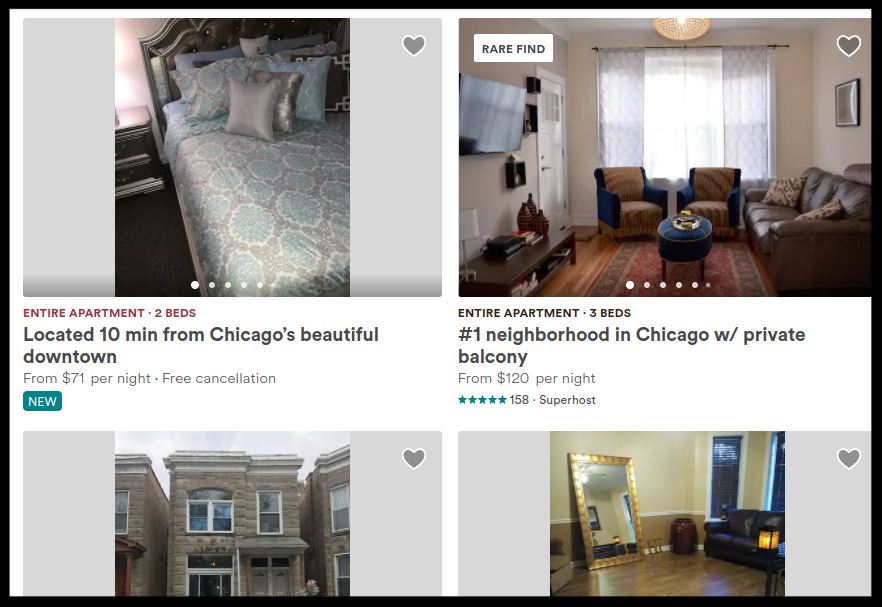This is a digital advertisement showcasing rental properties. 

To the left, there is an image of a bedroom. The bed, which is quite large, is adorned with numerous pillows, some featuring satin pillowcases in shades of silver and blue. The bedsheets are a mix of brown and turquoise hues. Next to the bed, there is a nightstand with a lamp, and the room has a brown carpet. The accompanying description reads: "Entire apartment with two beds, located just 10 minutes from Chicago's beautiful downtown, available from $71 per night. Free consultation included."

On the right, there is an image of a living room. It features a large brown leather couch and two chairs placed side by side, one brown and one blue. The description reads: "Entire apartment with three beds, located in the number one neighborhood in Chicago, featuring a private balcony. Available from $120 per night. Rated 158 stars."